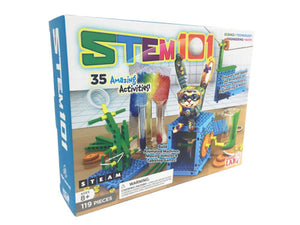This image depicts a STEM educational product targeted at children aged 8 and older. The product, titled "STEM 101," includes 119 pieces and advertises 35 amazing activities. The set is reminiscent of Lego in appearance but features unique plastic connections allowing for the assembly of various objects. The box, primarily white with a blue border, prominently displays the colorful "STEM 101" title, with letters transitioning from green to blue, purple, and pink or red. The visuals on the box feature blue, green, yellow, and red parts that can be assembled. Centrally positioned in the image, the box highlights the different projects that can be built, creating a vibrant and engaging educational tool focused on STEM topics.